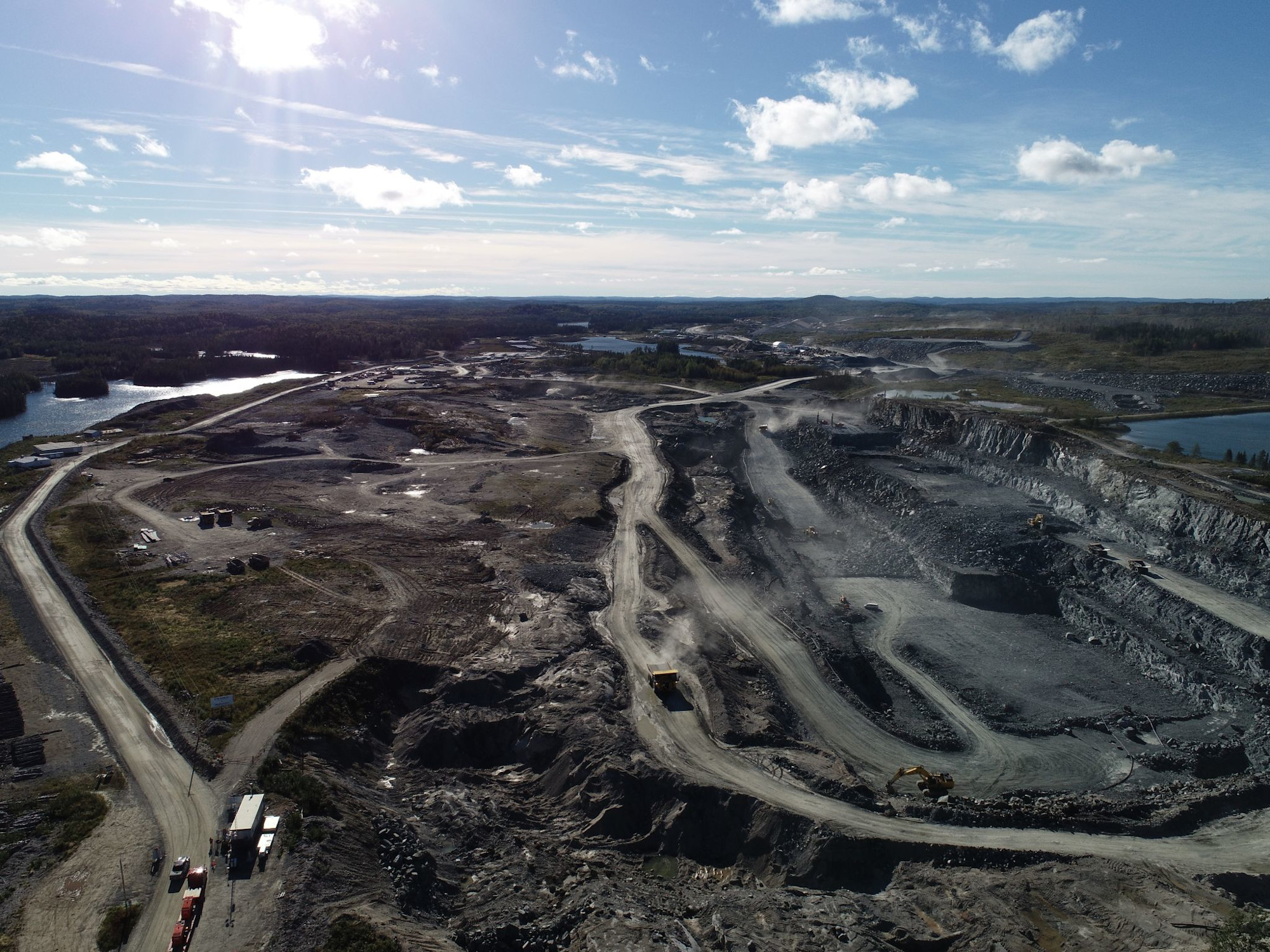This aerial image captures a sprawling, flat landscape featuring a mining operation. The Sun is partially obscured by a cloud in the upper left, casting a muted light over the scene. The sky is dotted with scattered small clouds, creating a picturesque backdrop. 

In the foreground, the land is crisscrossed with dirt roads and tracks, some of which arc and fork through the area. One prominent dirt road curves around the left side and forks towards the center, connecting to various sections of the site. Small cliffs and stepped levels are visible, indicative of active mining activities. The terrain is predominantly stripped and excavated, with several patches of exposed, dark soil.

Several bodies of standing water punctuate the dry landscape. These include a noticeable water body to the left, another on the right, and a central one in the distance. The water bodies could be natural lakes or man-made retention ponds designed to manage water flow within the mining area.

A variety of vehicles populate the lower left quadrant: three red vehicles that might be linked, a dark one traveling in the opposite direction, a long bus-like or semi-truck vehicle, and a shiny object that could be either a small vehicle or machinery. Additionally, a construction vehicle with an arm and scoop, and another resembling a dump truck, are situated on the right.

The horizon stretches far into the distance, adorned with distant trees, beyond which the deep blue sky and white puffy clouds dominate the upper expanse of the image. The scene reflects a dynamic blend of industrial activity and natural elements, unified under the bright, partially cloudy sky.